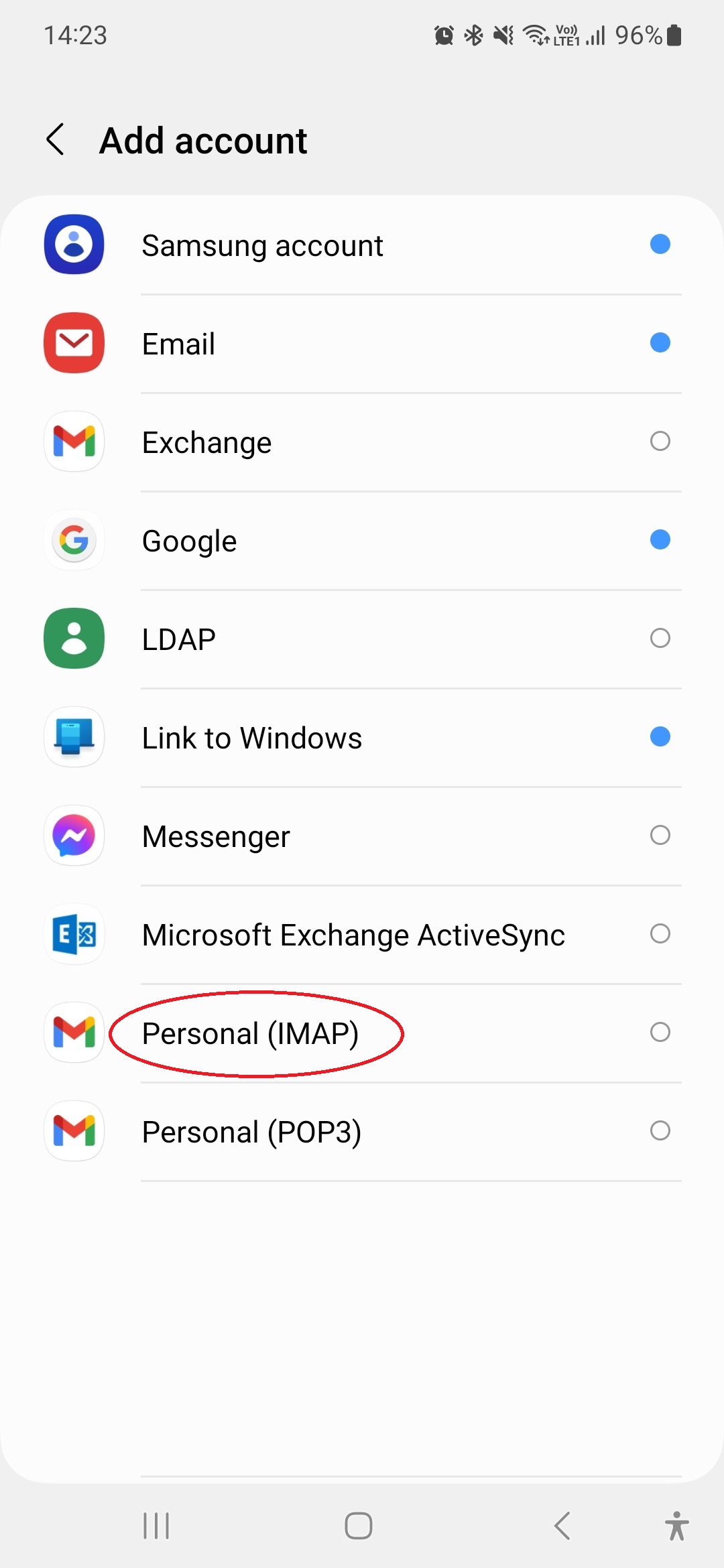The screenshot showcases a cell phone interface with a prominent gray bar at the top, where the current time is displayed in the upper left corner, alongside various status icons on the right. A left-pointing arrow shaped like a sideways "V" appears about three lines down on the left side. To the right of this arrow, bold black text reads "Add account." 

Below this header, a list of account types is presented, each within a white rectangle. Every type has an associated icon on its left, a name in the center, and a clickable circle on the right. Some circles are filled blue, indicating selection, while others are outlined in thin gray lines, indicating non-selection. 

The list of accounts includes:
1. **Samsung account** - The circle is blue.
2. **Email** - The circle is blue.
3. **Exchange** - The circle is unclicked.
4. **Google** - The circle is blue.
5. **LDAP** - The circle is unclicked.
6. **Link to warehouse** - The circle is blue.
7. **Messenger** - The circle is unclicked.
8. **Microsoft Exchange ActiveSync** - The circle is unclicked.
9. **Personal (IMAP)** - The circle is unclicked.
10. **Personal (POP3)** - The circle is unclicked.
11. **Personal IMAP** - The circle is highlighted with a red oval.

At the bottom, there appears to be extraneous text which may relate to a file type: "Microsoft Word 97-2003 Document MSWordDoc Word.Document.8."

This image likely serves as a visual representation of account settings within a mobile device.